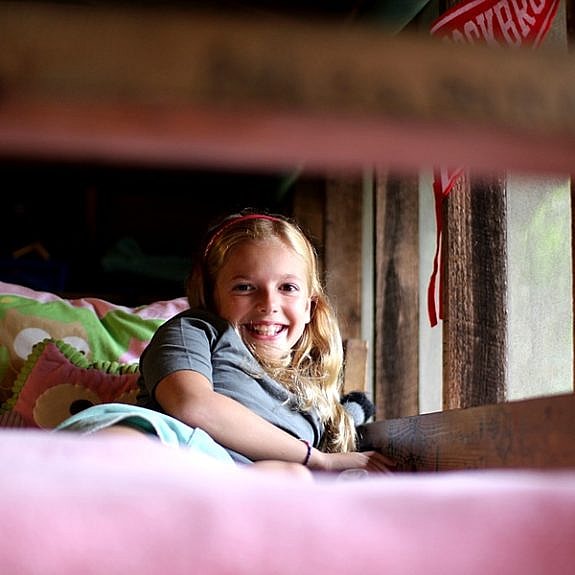In this photograph, a young girl, approximately 12 years old, lies in her wooden bed, smiling broadly with an open mouth as she looks directly at the camera. She has long, very blonde hair adorned with a red ribbon. She is wearing a grey short-sleeved t-shirt and light blue shorts or a skirt. Her bed is covered with pink sheets and is decorated with cartoon figures on the throw pillows, including one with a large white eye and pink and green edging. The girl's right hand, draped across her chest, has wrist jewelry. Behind her, frosty and misty windows suggest it may be raining outside. Above the window, a red college pennant with white lettering hangs, though the text is obscured in the photo.